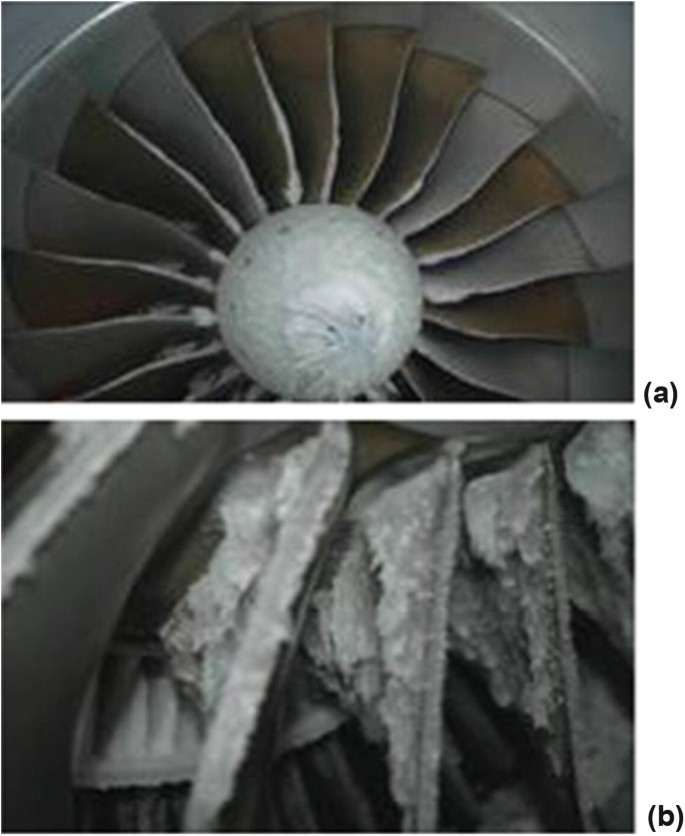The image is divided into two sections, with the top image (A) showcasing a close-up of a turbine or airplane engine. This part of the engine features approximately 20 to 30 metallic fan blades arranged in a circular pattern around a central bolt, with the entire assembly being predominantly silver and dark gray. The bottom image (B) provides an even closer look at these fan blades, revealing significant buildup on their surfaces. This buildup, which could be ice, dust, or mineral deposits, heavily coats the blades, indicating they have accumulated substantial residue over time. The image collectively illustrates the contrast between the structural integrity of the turbine and the operational wear affecting the blades.